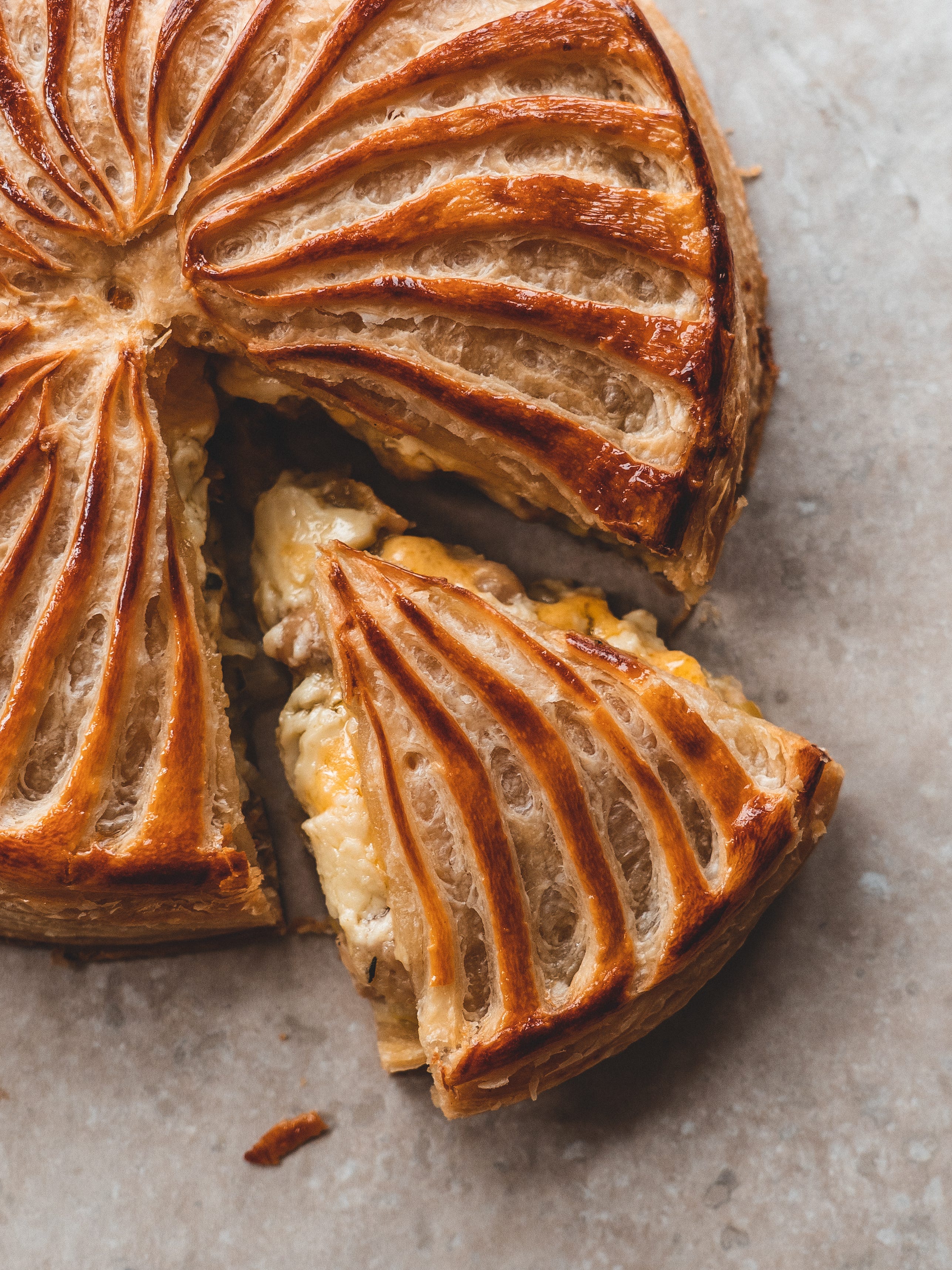The image showcases a partially sliced pie, presenting a golden-brown crust that's been brushed to achieve a crispy texture, particularly along the patterned streaks. The pie is centrally positioned on a light brown, granite-like countertop, emphasizing its rustic appeal. A slice has been taken out and slightly separated from the whole, revealing a tantalizing glimpse of its bubbling, possibly savory filling, which includes elements that could be cheese, meat, or even a blend of both. Crumbs from the pastry sprinkle the surrounding area, enhancing its homemade allure. Although the pie's exact ingredients remain indistinct, the combination of golden and brown hues with streaks of white and yellow hints at a rich, hearty composition.